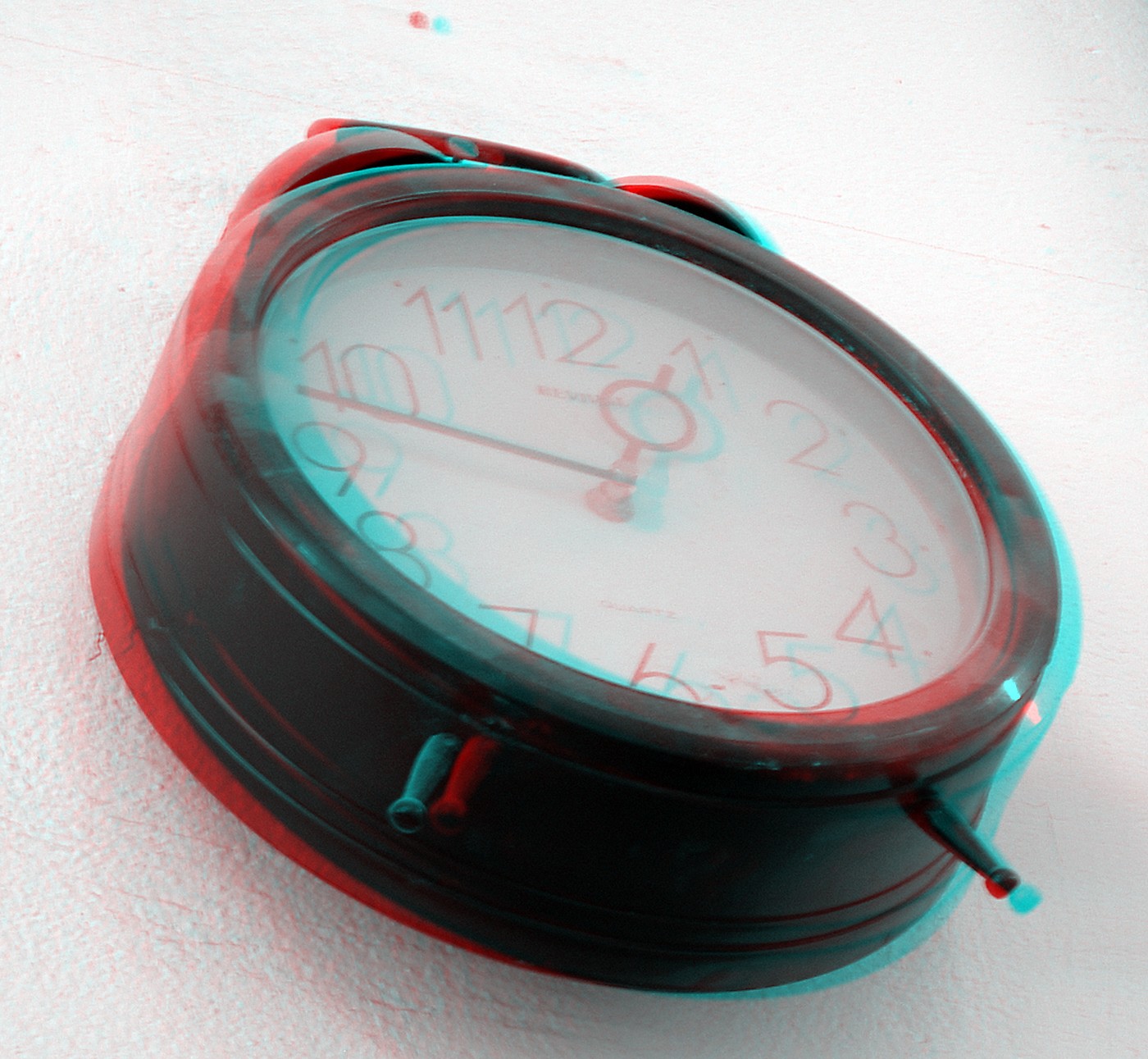This photograph features an old-fashioned, retro-style analog alarm clock set against a white background. The clock is designed with small legs at the bottom, two little bells, and a handle on top, giving it a classic, nostalgic appearance. The clock's face is marked with white numbers and showcases red hands, indicating the time is approximately 12:50 or 12:55. The clock body appears black, but it’s enhanced with a pop art filter, giving it a striking, holographic effect with vivid red and blue hues. These contrasting colors create a visual impression of the clock shaking or having a double-vision, ghosted appearance, adding to the dynamic and artistic feel of the image. The edges of the clock and the numbers seem to blur and shift due to this effect, making the entire piece appear animated and vibrant.